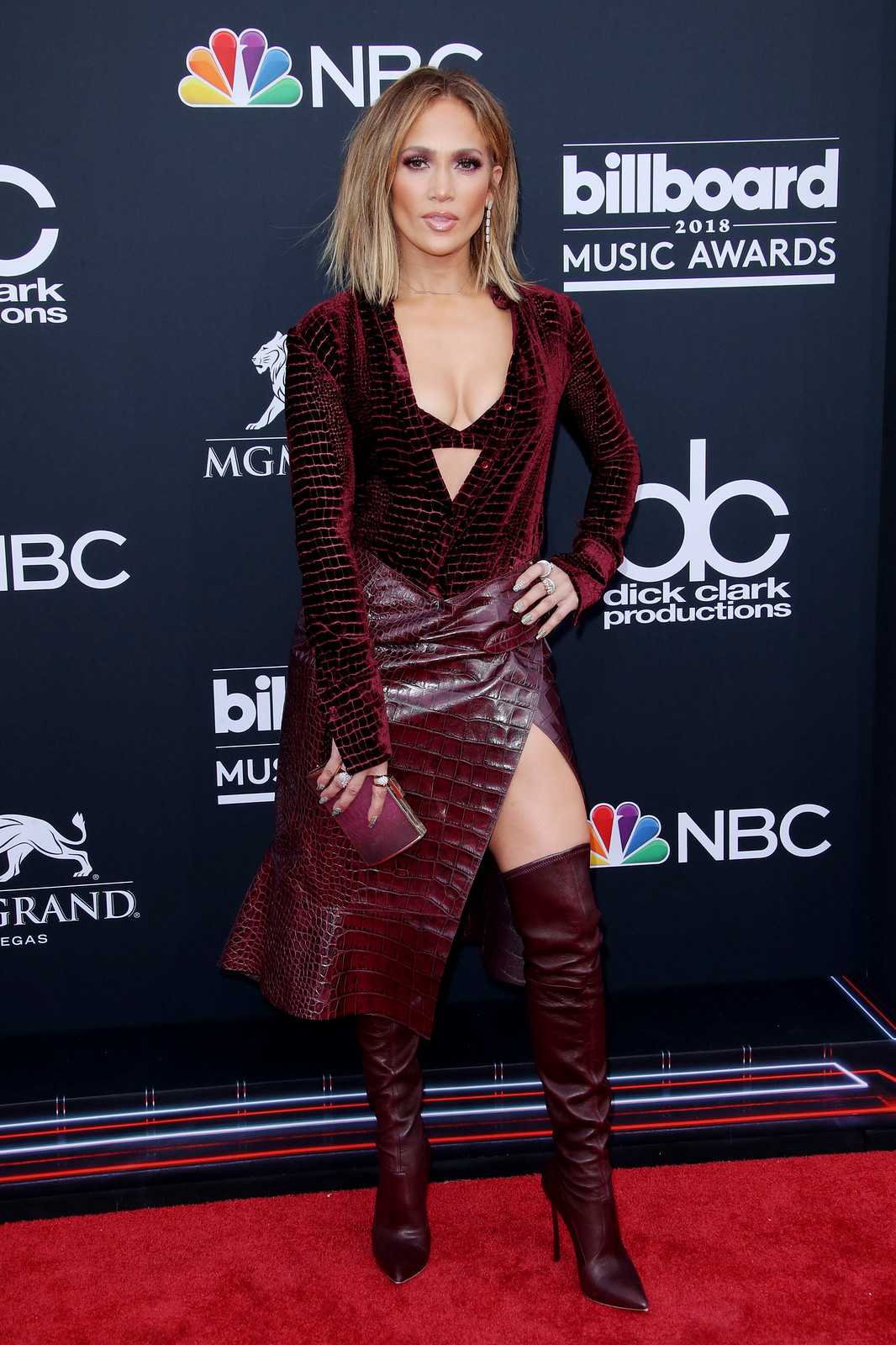In this detailed photograph, Jennifer Lopez is seen on the red carpet at the NBC Billboard 2018 Music Awards, produced by Dick Clark Productions. The backdrop is a dark gray screen adorned with multiple logos, including the NBC peacock, Billboard, and mentions of Las Vegas. Jennifer Lopez, often known as Jenny from the block, exudes glamour with her shoulder-length blonde-brown hair styled in a long bob. She is dressed in a striking ensemble comprising a velvety maroon bra, a matching long-sleeve blazer, a high-slit maroon leather skirt, and thigh-high maroon leather boots. Her sophisticated look is complemented by earrings, and she is confidently posing for the camera. The red carpet beneath her and the colorful NBC logo add vibrant hues to the overall scene.